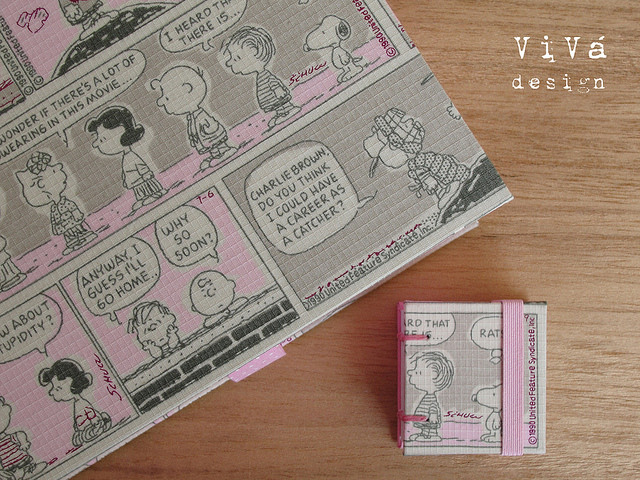The image is of a partially cut-off Peanuts comic strip displayed diagonally on what seems to be a desk with a wood-tone background. The comic strip features Sally asking Lucy and Charlie Brown, "I wonder if there's a lot of swearing in this movie," to which Linus replies, "I heard there is." The subsequent panels include Lucy saying, "How about stupidity?", Linus mentioning, "Anyway, I guess I'll go home," and Charlie Brown responding, "Why so soon?" Another panel shows a character asking Charlie Brown, "Charlie Brown, do you think you have a career as a catcher?" Part of the comic strip is folded and secured with a pink rubber band-like substance. The colors in the image are predominantly black, white, gray, pink, and brown. In the lower right-hand corner of the image, the text "Viva Design" is visible in white. Additionally, small, unreadable text appears on the side, and elements such as the word "Schultz" and characters like Snoopy and Linus are also included.